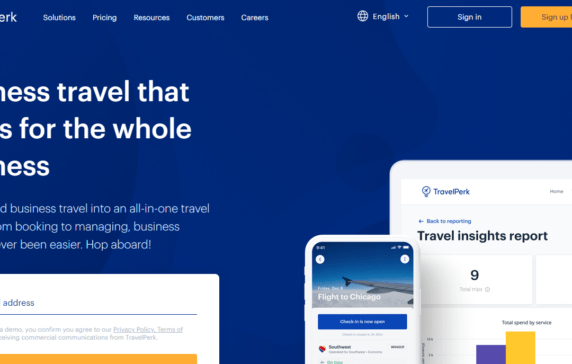This screenshot captures a partially visible website with a royal blue background. The upper section features white text, with the truncated website name "ERK" on the left. Adjacent to this, a horizontal menu offers options labeled Solutions, Pricing, Resources, Customers, and Careers. Toward the right side of the menu is a language selection drop-down, currently set to English, followed by two buttons: a gray "Sign In" button and a prominent yellow "Sign Up" button.

In the main body of the website, white, partially-obscured text dominates the royal blue backdrop. Visible text includes "Ness Travel," missing the initial "S" in "Ness." Below this header, smaller white font reads, "Business Travel into an all-in-one travel. I'm booking to managing business. Verb in easier. Hop aboard." Directly beneath this text, there is an input field for entering an email address, with a stylized graphic of a non-realistic smartphone to its right. This combination of elements suggests a user-friendly interface aimed at facilitating business travel management.